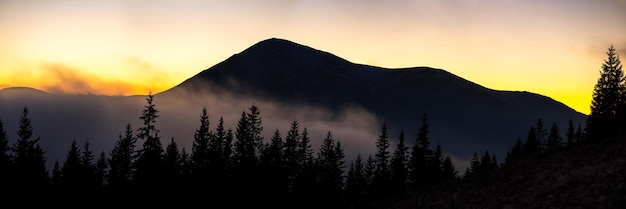A breathtaking panoramic photograph capturing the serene beauty of a mountainous region at dawn or sunset. The image spans wide horizontally, offering an expansive view while being shorter vertically. Along the darkened silhouette of the mountain range, the sky glows with stunning golden hues, transitioning into lighter yellows and grays as it ascends. Below the majestic mountains, a line of pine trees stretches from left to right, standing in a near-straight formation. A thick layer of fog lies close to the ground, blanketing the area between the trees and the mountains with a soft, powdery appearance, adding an ethereal quality to the scene.